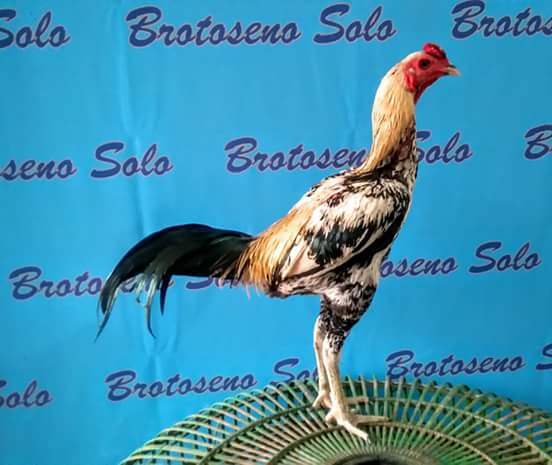In this detailed image, we see a small, thin rooster with distinct coloration standing on what appears to be a light green and rusted circular metal table or possibly a fan turned on its side. The rooster, which is facing to the right, has a striking red face and a long neck with yellowish-orange feathers on the back, transitioning to black and white spotted feathers on the underside and across its chest and wings. The bird has pure white legs and a black tail, with a touch of orange and yellow on its back before the tail feathers. In the background, there is a light blue banner with repeated text in darker blue that reads "Brotacina Solo." The banner provides a soft, monochromatic backdrop that highlights the vibrant hues and intricate details of the rooster.